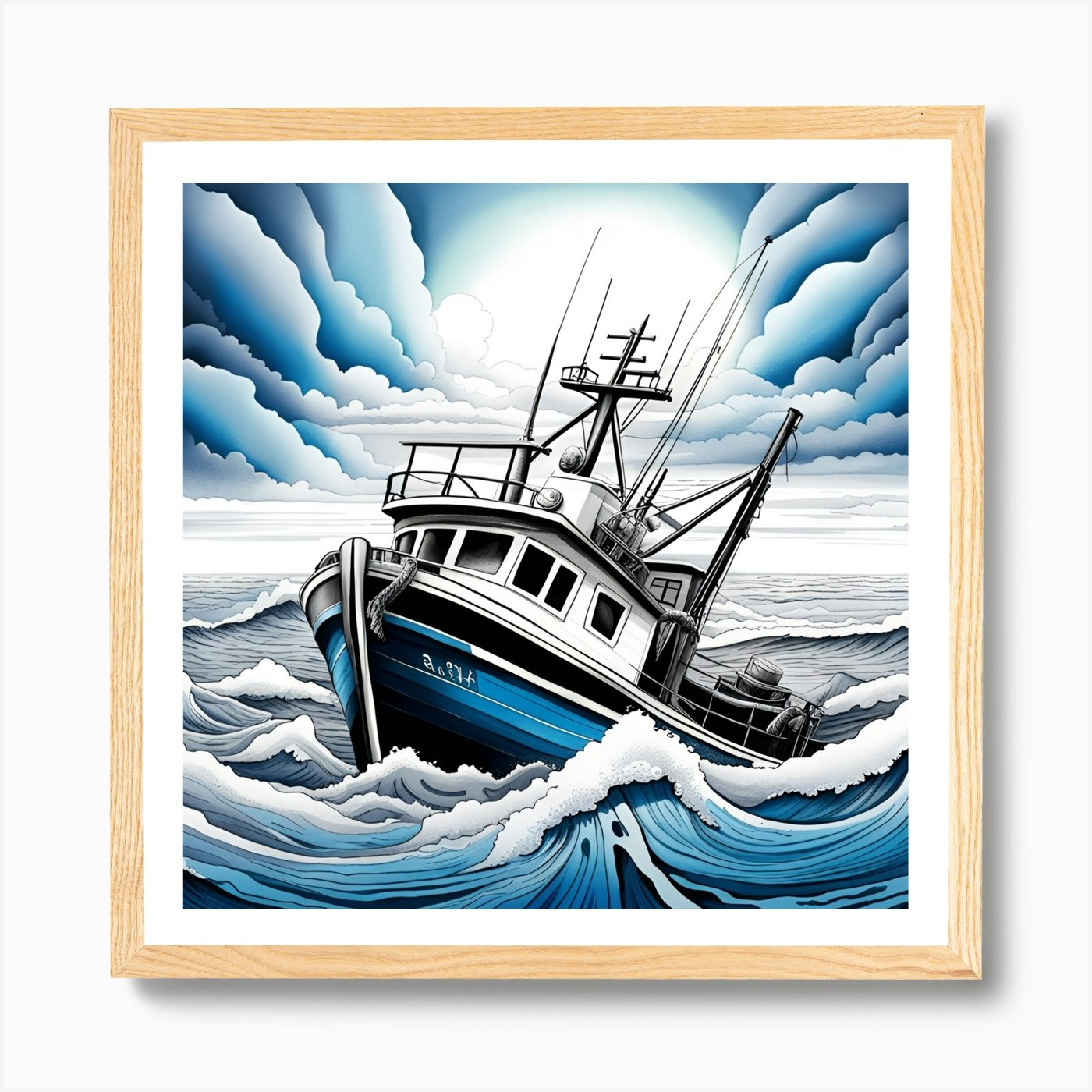The image portrays a small blue and white fishing vessel being violently tossed in extremely rough seas, identifiable by the numerous rods, reels, and antennas on board. The ocean is tumultuous, with large, crashing waves capped with frothy white foam, indicative of severe and active waters. The sky above is dark and stormy, though there's a faint light turquoise glow at the center, suggesting a parting of the clouds. The boat appears sideways, suggesting it is being thrown around by the powerful waves, which break higher in the background. Framed in wood with a white and ivory matting, the scene captures a dramatic maritime struggle with no calm waters or people in sight.